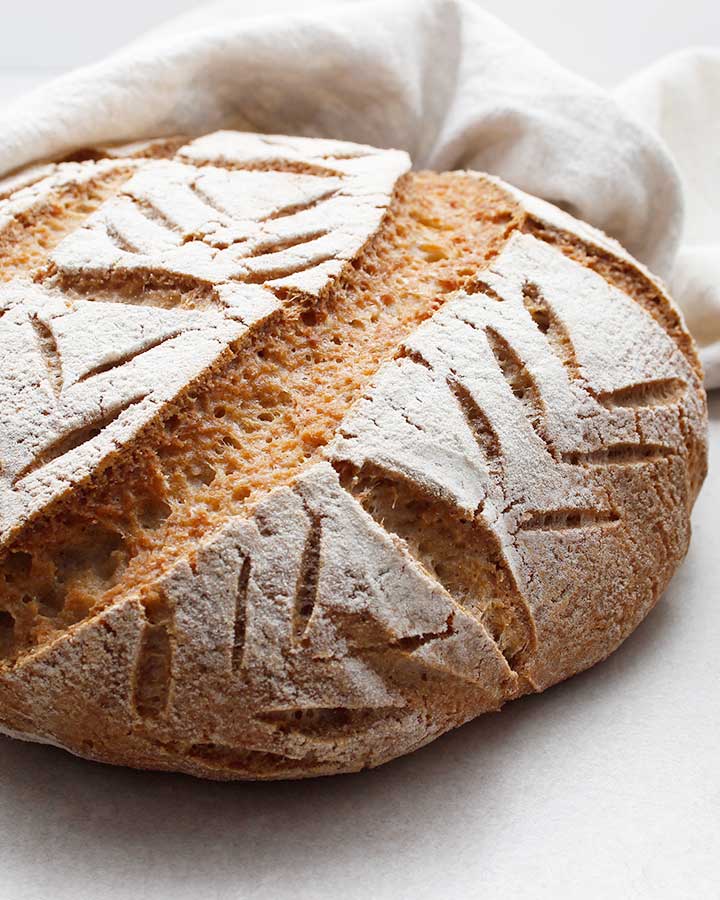This is a close-up image of a loaf of homemade bread, showcasing its rustic and artisanal qualities. The bread's crust is predominantly covered in a white flour dusting, which contrasts with its light brown surface. The loaf is divided into three main sections by subtle indentations that run parallel to its crust, giving it a textured appearance. Notably, the crust features a decorative pattern of three V-shaped marks grouped together, with a horizontal line bisecting the loaf and another set of V-shaped marks below it, resembling arrows pointing downward. The bread sits on a white cloth and rests on a gray platform, with a soft shadow cast beneath it, suggesting it may have just been pulled from the oven to cool. The overall texture varies, presenting both rough and smoother areas, adding to its appealing, handmade aesthetic.